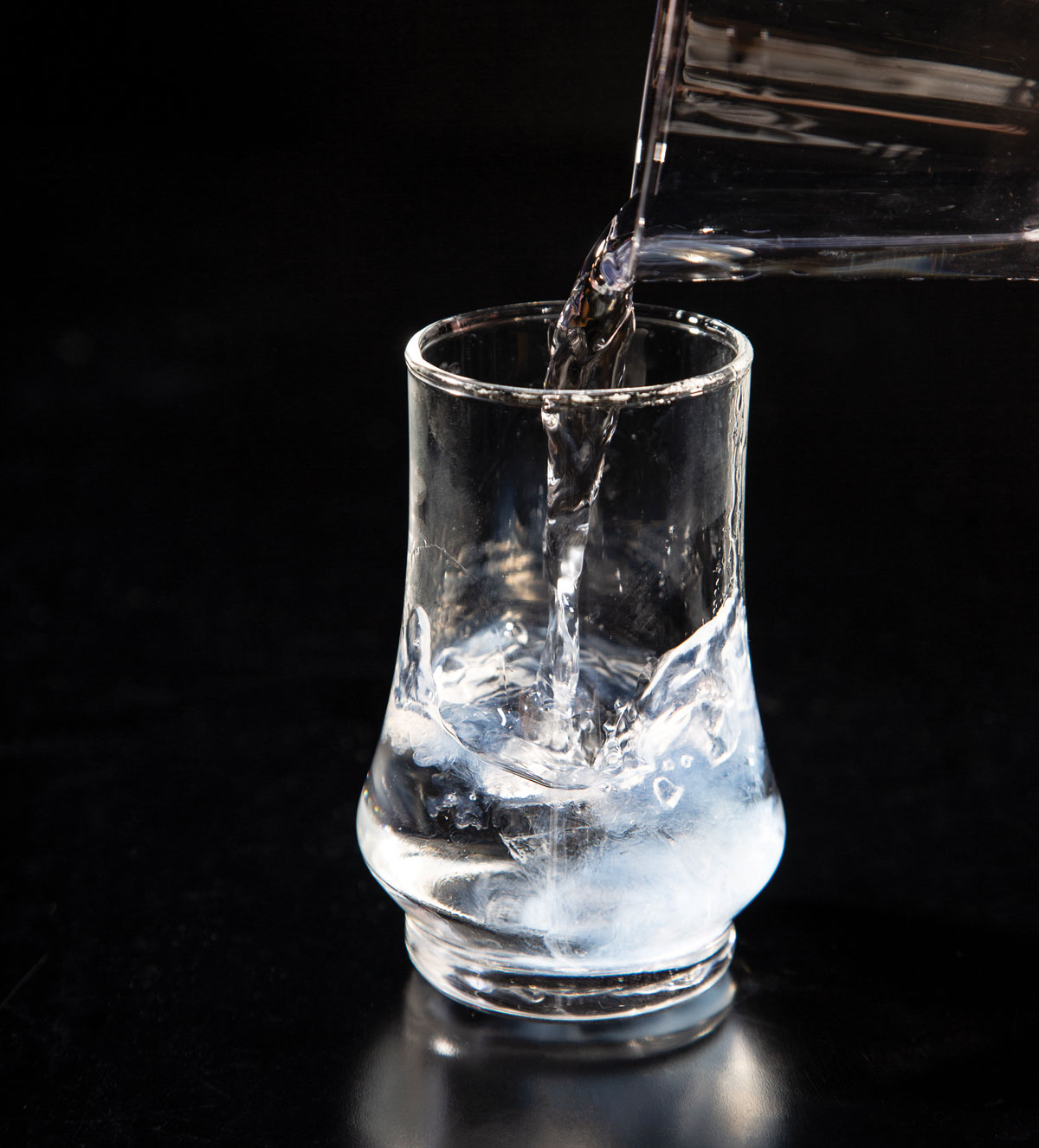This professional photograph features a glass cup being filled with water, captured mid-pour. Both the pouring container and the glass cup are made of glass. The scene is set against a stark black background, which highlights the clarity and design of the glassware. The glass, positioned on a highly reflective black surface, displays a vivid reflection of itself in the foreground. 

The glass cup has a distinctive shape: a wide bottom tapering inward at the middle, then flaring slightly outwards to a narrower, chimney-style top. It stands on a narrow, round glass pedestal beneath its widest part. The cup is halfway filled with clear liquid, which appears frothy, suggesting either water or a mixed drink, potentially with ice cubes—though this is obscured by the froth. 

The liquid is being poured from another glass container on the right side of the frame, held at a perpendicular angle to the upright glass cup. The absence of text or additional elements focuses attention entirely on the elegance and design of the glassware and the dynamic motion of the pouring water against the minimalist black background.